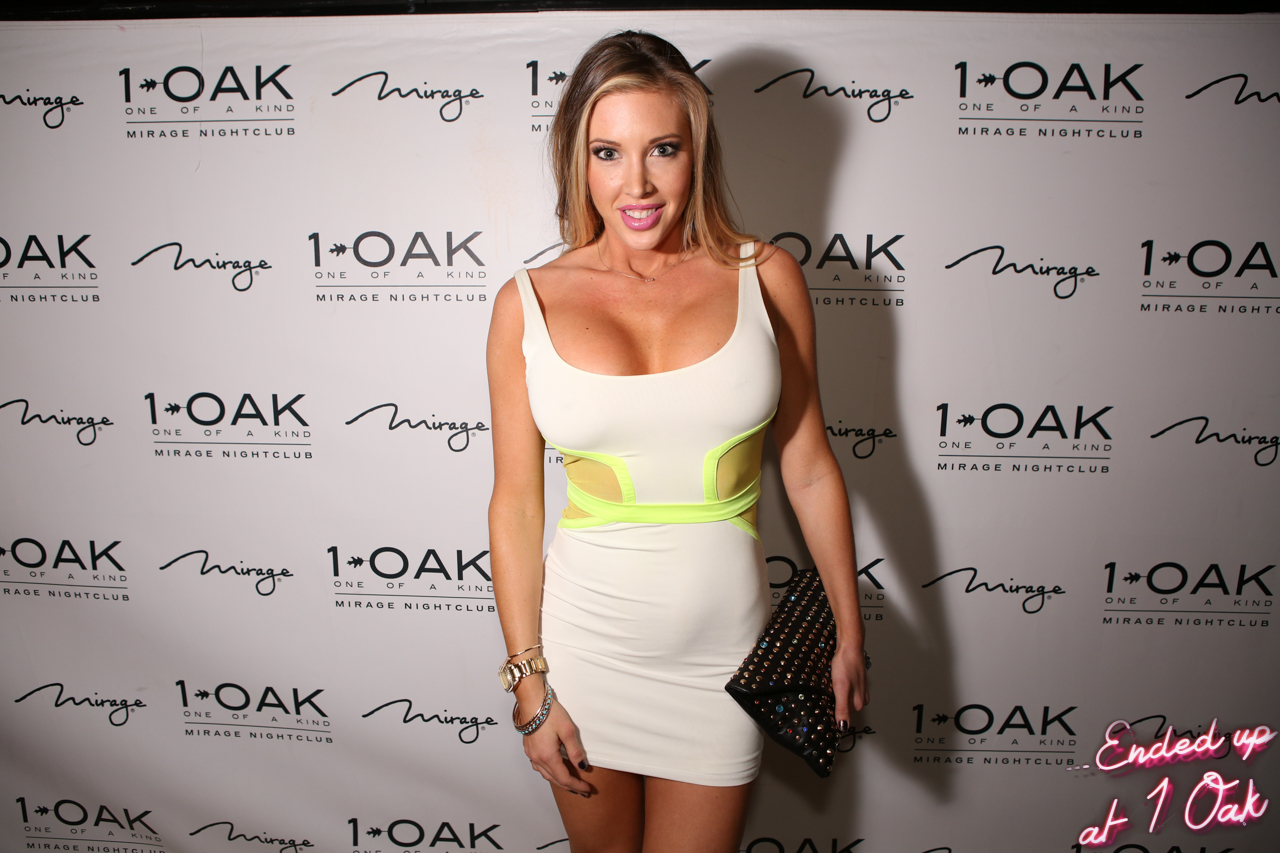A detailed photograph captures a smiling, voluptuous white woman with long blonde hair and blue eyes, standing confidently in front of a white backdrop adorned with various logos for One Oak and Mirage Nightclub. She is wearing a strikingly short, tank-top-style white dress with yellow accents, featuring both a yellow belt and cut-out sides that reveal her skin. The dress leaves her upper thighs and much of her cleavage exposed. She accessorizes with a black clutch bag adorned with rhinestones, held in her left hand, and sports bracelets and a watch on her right wrist. Her nails are painted dark, and she is wearing pink lipstick and mascara. The backdrop includes multiple One Oak and Mirage logos, with the phrase "Ended Up at One Oak" prominently displayed in bright pink neon letters in the lower right corner. The main focal point of the image is the woman standing in the center, exuding confidence and style.